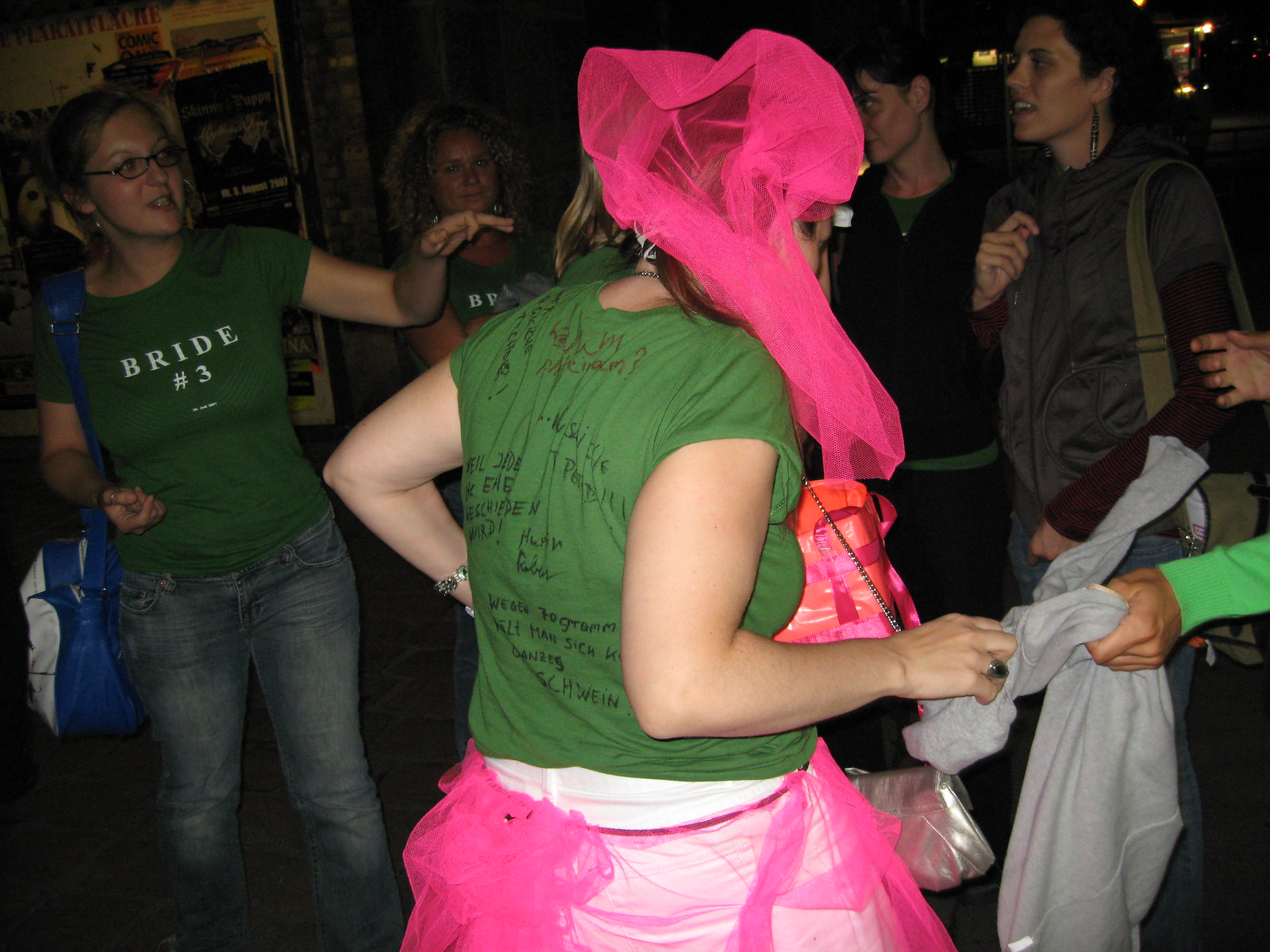The photograph captures an exuberant bachelorette party taking place outdoors at night. The central focus is on a woman facing away from the camera, clad in a green T-shirt covered in handwritten signatures and slogans. She sports a vibrant pink veil and a pink tutu over white shorts, complemented by a shiny silver purse slung over her shoulder. Surrounding her, other partygoers are visible, including a woman on the left pointing with a blue and white duffel bag and glasses, also wearing a green T-shirt emblazoned with "Bride No. 3." Another woman, similarly dressed, chats in the background. The scene, bustling with energy, suggests a lively celebration likely held at a nightspot adorned with posters.